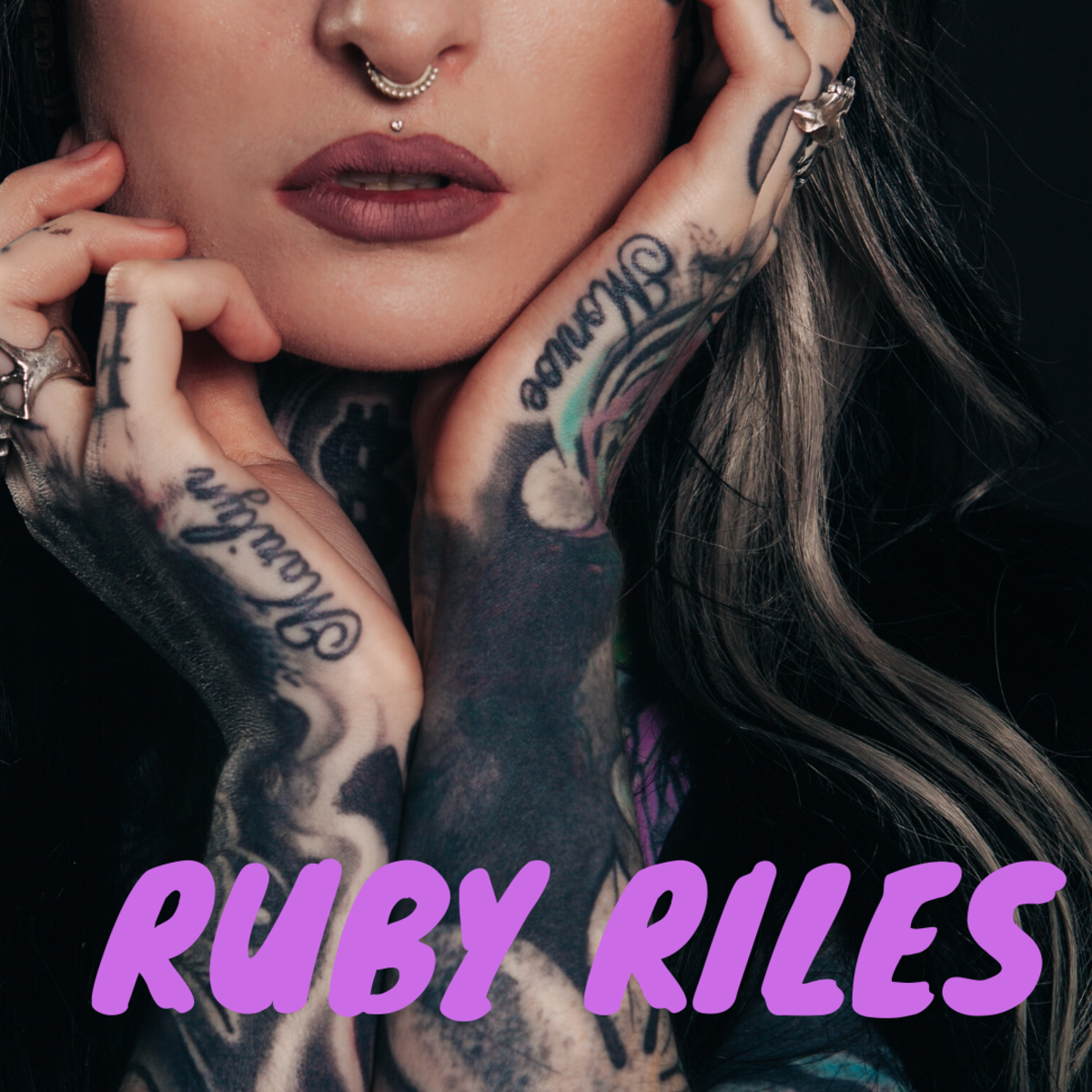This vertical rectangular promotional image prominently features Ruby Riles, whose name is displayed across the bottom in large purple letters. Behind the text, there is a close-up photograph of a woman, visible only from her upper shoulders to just below her nose, excluding her eyes entirely from the frame. She has very long hair and both her hands are dramatically cupping her face, revealing intricate tattoos that cover her fingers, the backs of her hands, and extend down her forearms. Among the tattoos, the words "Marilyn" and "Monroe" are distinctly inked on the sides of her hands. She sports a metallic red lipstick, a nose ring adorned with gems, and a lip piercing, adding to her edgy aesthetic. The woman is wearing a black top, blending slightly into the black background which gives the impression that she is emerging from a dark void. Overall, the image is detailed with colors including black, brown, tan, purple, light blue, and dark red, and it seems to be crafted in a way that emphasizes its primary subject, likely portraying Ruby Riles in a modern, stylized manner befitting a celebrity or model.